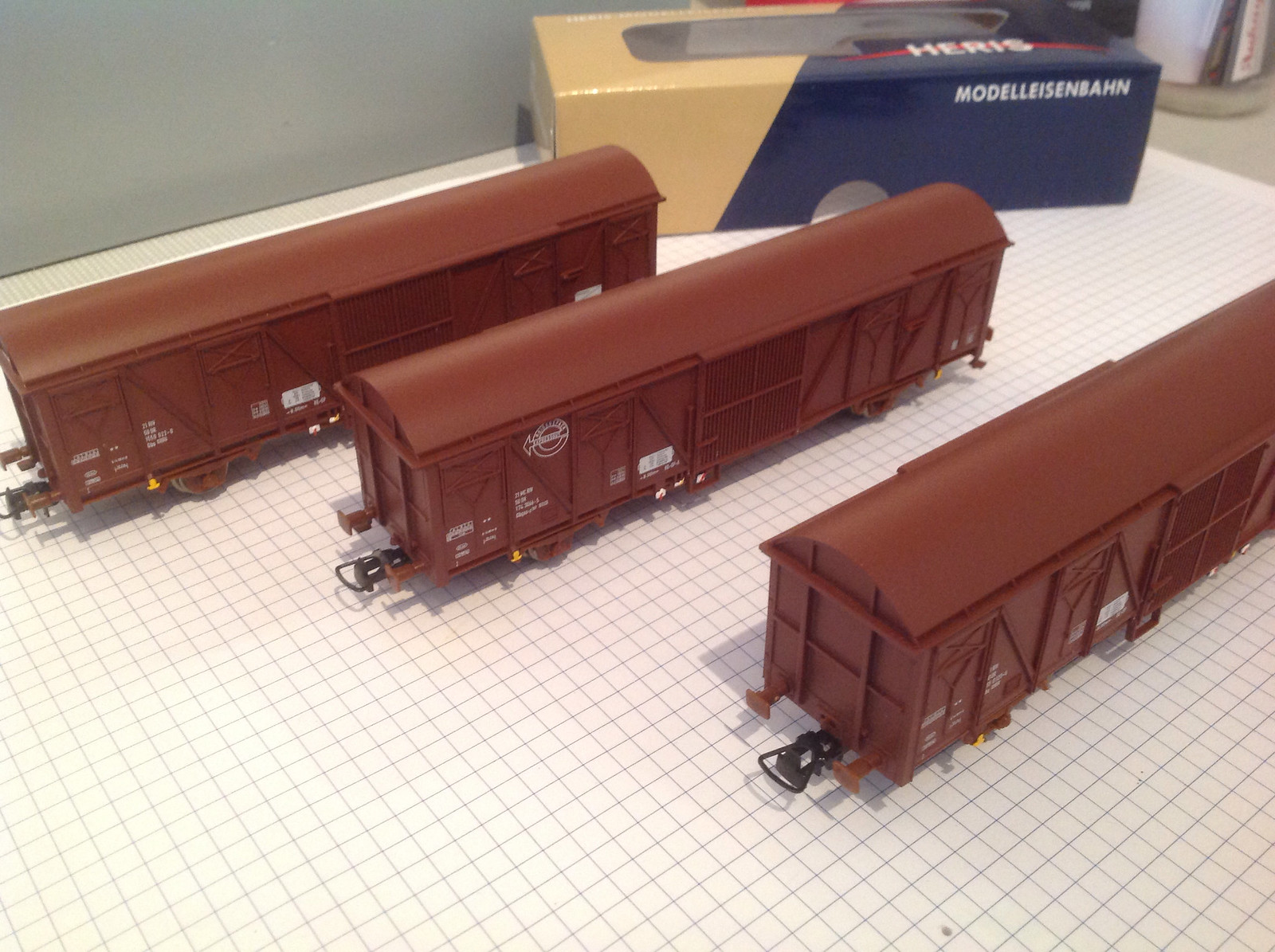This detailed photograph captures three identical model train box cars positioned on a tabletop covered with white paper featuring a grey grid pattern. The box cars, made from a plastic material, exhibit a dark reddish-brown to burgundy hue with intricate details, including small white logos and print that are too fine to decipher. Each car is equipped with black couplings at the front. In the background, there's a blue and yellow diagonally split box with a red-lined logo spelling "HERIS" in white, and additional text "Modelleisenbahn." The scene is set against a wall of muted greenish-grey color, enhancing the meticulous setting of this model train display.